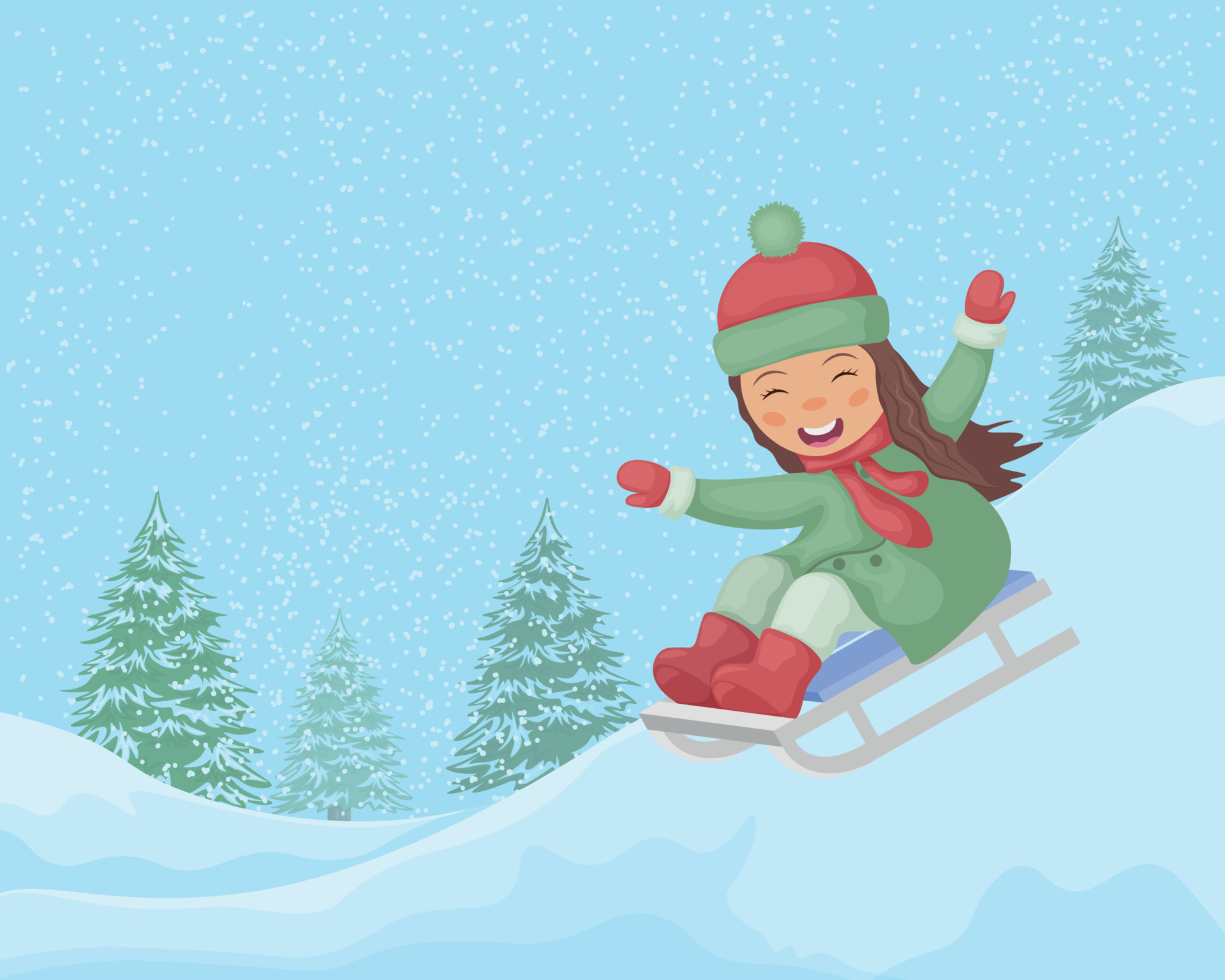A joyful girl, reminiscent of clip art, is depicted sledding down a snowy hill. Her long, brown hair cascades past her shoulders as she smiles and laughs exuberantly. She rides a blue sled with gray blades, gliding over snow that has a light blue tint extending across the image. Her happiness is palpable as she enjoys the wintry adventure. The girl wears bright red mittens on either hand and a matching red hat. Perched atop her head is a small green accessory, possibly a button or decorative pow-wow. In the background, snow-covered trees add a serene, wintry touch to the vibrant scene.